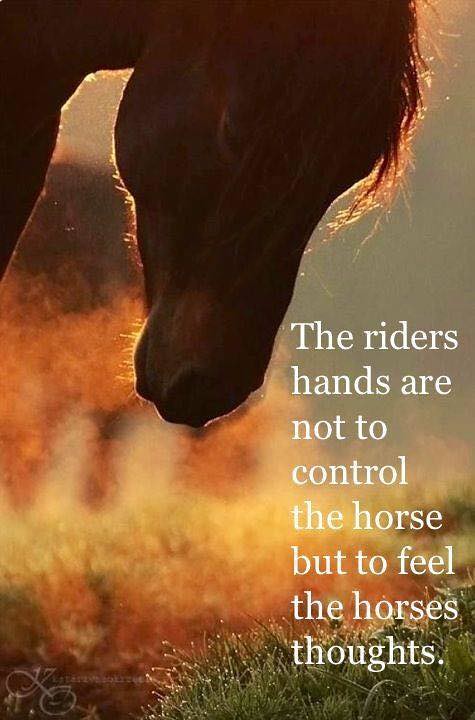The photograph captures a serene brown horse with a dark mane, its head bowed towards the dew-covered, green and gold grass. The horse's tuft of hair hangs down over its forehead, and its open eyes are faintly visible. The sunlight behind the horse casts a gentle illumination, possibly indicating early morning or late afternoon—sunrise or sunset—enhancing the golden brown and black leaves of a distant tree. An inspirational quote in white font runs vertically along the right side of the image, stating, "The rider's hands are not to control the horse, but to feel the horse's thoughts." The background showcases a blend of muted burnt orange and yellow hues, adding a warm, autumnal essence to the scene. An indistinct image, possibly a bike symbol, appears etched in the lower-left corner, contributing a subtle, postcard-like charm.